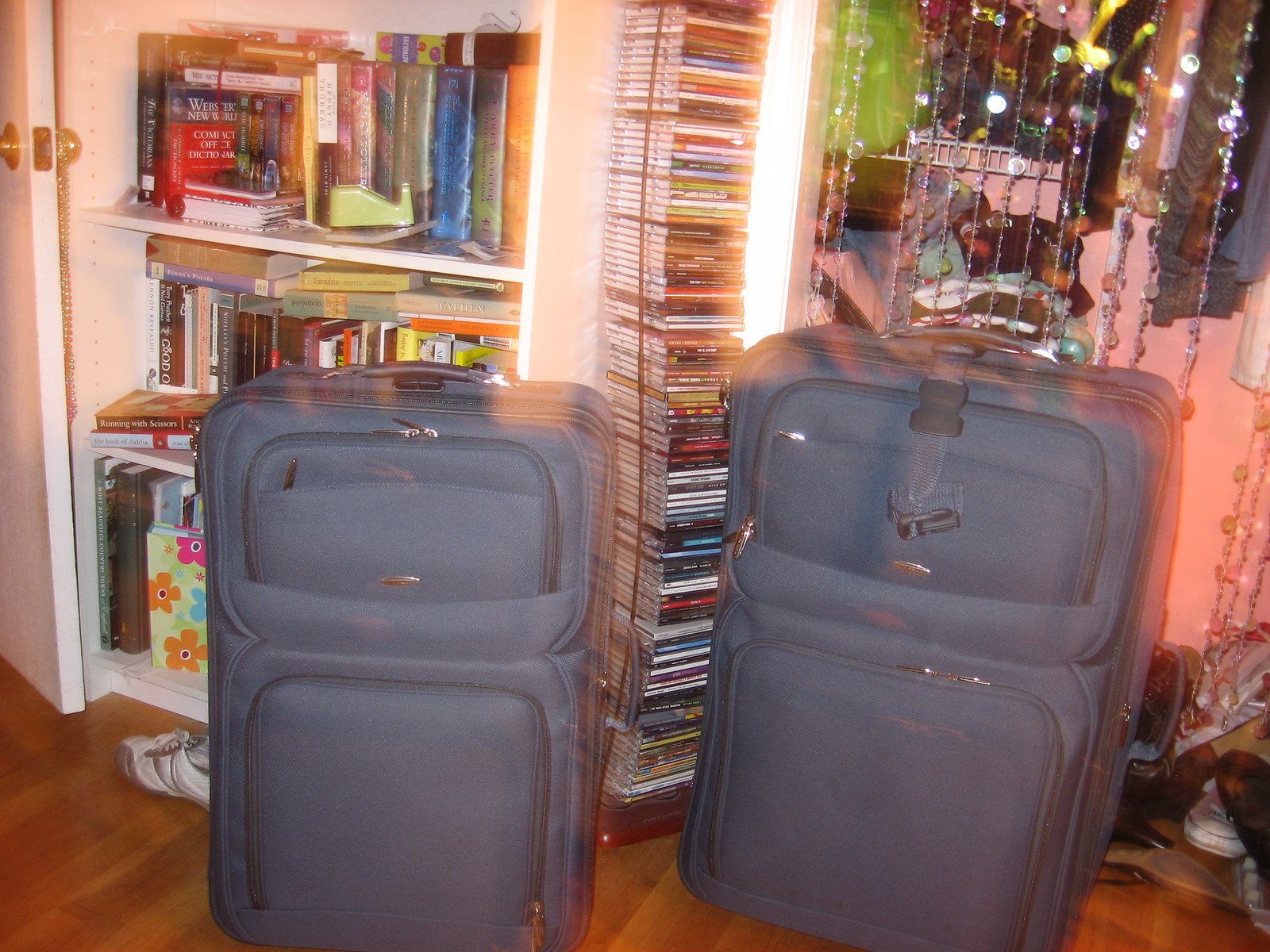This indoor photograph captures a cozy room with an eclectic ambiance. Dominating the foreground are two large cloth suitcases, one slightly smaller than the other, both appearing dark in color—either black or dark blue. They are placed on a medium tannish brown hardwood floor, with pairs of shoes flanking the suitcases on both the left and right sides of the frame. 

In the background, a pinkish-toned wall provides a warm contrast to the various elements in the room. On the left side, a white bookcase with three shelves is filled with an array of books, though the titles are not discernible. Next to the bookcase, a door is partially visible. The right side of the image reveals a closet with clothes hanging, partially obscured by semi-transparent or pink beaded curtains that dangle from the ceiling. Between the bookcase and the closet stands a tall tower of compact discs or DVDs, stored in a clear casing, adding a touch of vintage charm to what seems to be a personal or music room. The lighting in the room is somewhat blurred, creating blotches that soften the overall scene.